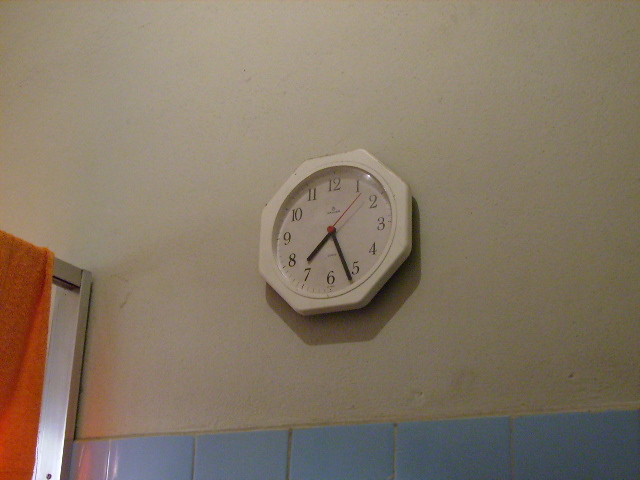The image features an octagonal white clock prominently hung on a primarily white wall with a slightly darkened hue. The clock, with its distinct octagonal shape encasing a circular face, displays the time as 7:26, with the minute hand slightly past 7 and the red second hand precisely at 8 seconds. The clock face is adorned with black numerals ranging from 1 to 12 and is covered with a clear glass or plastic protector. The top of the clock appears slightly dirty, marked with a brownish residue. Below the clock, the wall transitions into baby blue tiles. On the left side of the scene, part of a metal frame indicating the edge of a shower area is visible, holding an orange towel draped over it. The overall setting suggests this is a bathroom, with soft light possibly seeping through a nearby window enhancing visibility.